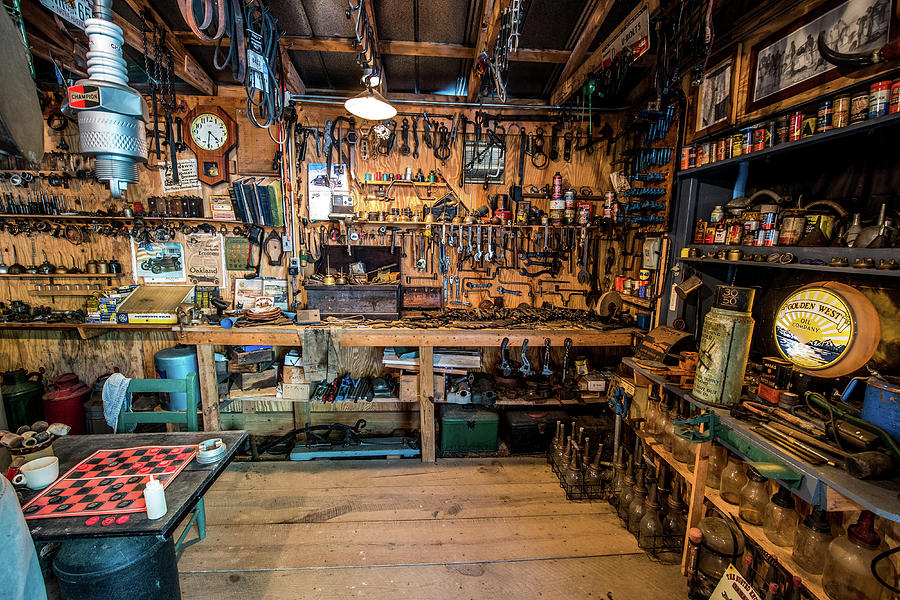The image depicts a rustic garage workshop with a plethora of tools displayed prominently on wooden brown walls. To the left of the scene, hanging on the walls and resting on shelves, is an extensive collection of tools including wrenches and various mechanic implements, as well as vintage oil cans, glass jars, and an old gas station globe. A wooden table is situated in the lower left quadrant, featuring a checkerboard top with three red checkers, a white coffee mug, and a white bottle with a spout. Nearby, a blue chair accompanies the table, while a green chair with a denim hat tossed over its corner sits opposite. Centered prominently in the upper left-hand corner, a brown wooden clock reads 4:32 PM. The floor is constructed of wooden slats, complementing the nostalgic, old-fashioned ambiance of the area which is reminiscent of a vintage general store. Scattered around the space, you also notice toolboxes and handyman essentials, hinting at the thorough and industrious nature of the workspace.